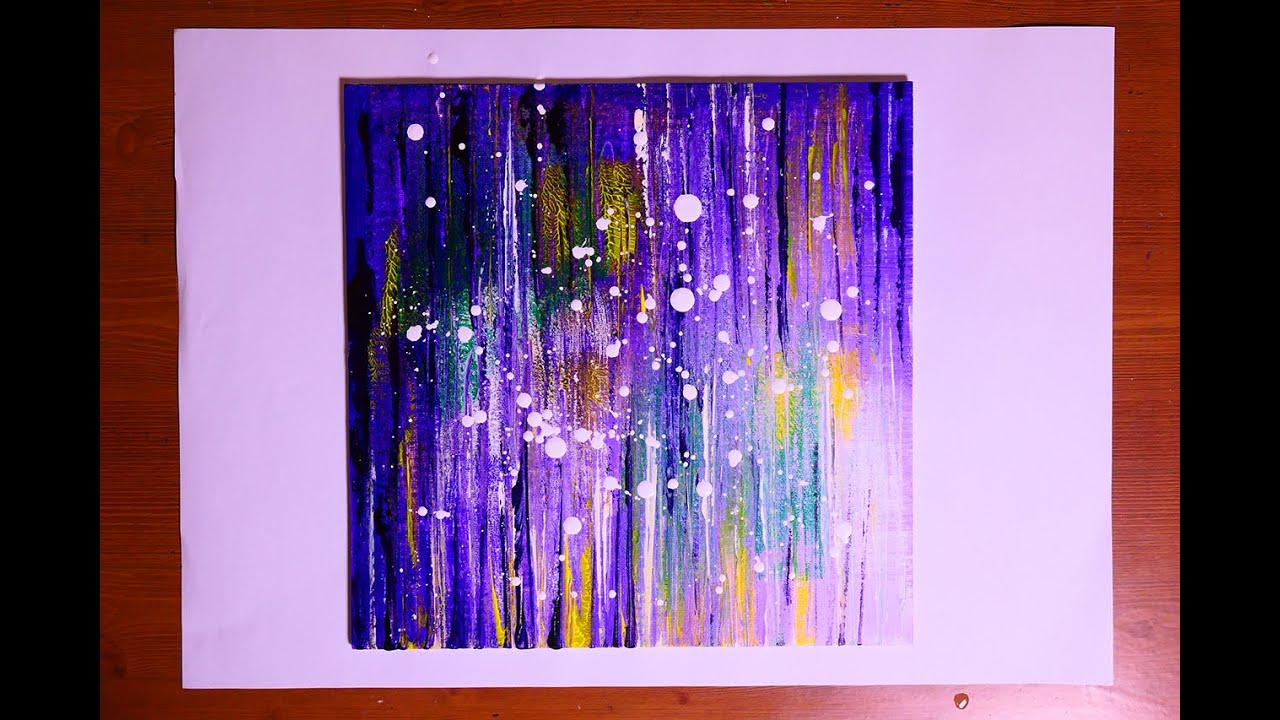This image depicts a detailed, modern abstract painting. The artwork, enclosed in a reddish cherry wood frame, is mounted against a white mat and appears to hang on a black wall. The main painting itself is a square composition showcasing vibrant, vertical streaks of colors—predominantly purple and blue, interspersed with gold, orange, yellow, green, and white. Various shades of each color are visible, adding depth and complexity to the piece. Scattered throughout the painting are white paint droplets of varying sizes, resembling snowballs against the vivid background.

Below and to the left of the painting, there are noticeable water droplets—the larger one situated at the bottom left and a smaller one near the top left corner. These droplets likely resulted from accidental splashes. The white mat around the painting not only emphasizes the central artwork but also has a stray droplet of paint in the top left corner, which seems incidental. Overall, this abstract painting harmonizes a multitude of vibrant colors and details, creating a dynamic and visually engaging piece.